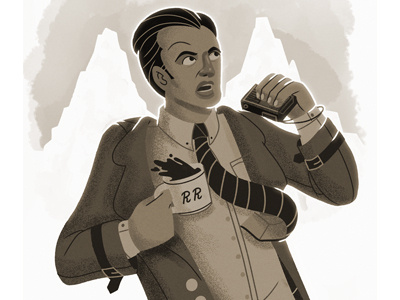The image is a black and white, comic book-style illustration of a man in a chaotic, rushed state. The man, who has dark slicked-back hair and visible sideburns, is dressed in a business suit complete with a white button-down shirt and a disheveled black-and-white striped tie. He holds a square, old-school handheld voice recorder in his left hand, raised to his mouth as if shouting something, and a white coffee mug marked with the black cursive letters "RR" in his right hand. The contents of the mug are noticeably spilling, indicating sudden movement. His facial expression signifies frustration or surprise, with his mouth wide open and his eyes turned to the upper left corner. The background consists of a stark white setting with gray shading, featuring a watercolor splash or smoke-like pattern coming from the top, and faint mountain-like formations can be seen. The overall depiction suggests he is hurried and agitated, emphasized by the chaotic positioning of his tie and the leather straps with silver buckles around the sleeves of his jacket.